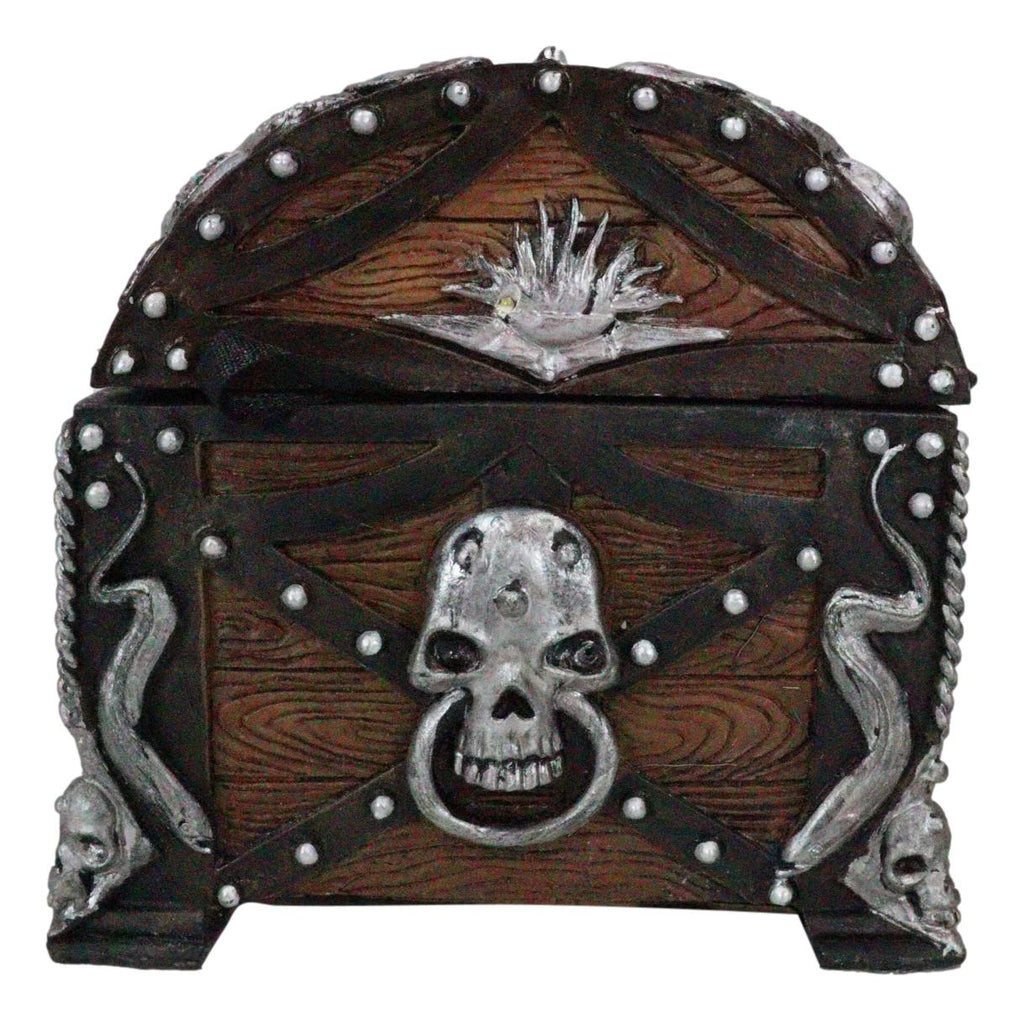The image depicts the side view of an intricately designed wooden treasure chest with a dark, rich finish and semi-circular dark patterns etched into the wood. The chest features a rounded top and a square base, all framed in robust metal trimmed with metal rivets. Central to the side panel is a striking silver artwork of a skull, with what appears to be a fiery torch above it. The sides of the chest showcase detailed silver images of a serpent coiling downwards, and smaller skulls are positioned near the corners. The embellishments add a dramatic and gothic flair, highlighted by the metal accents and their intricate designs.